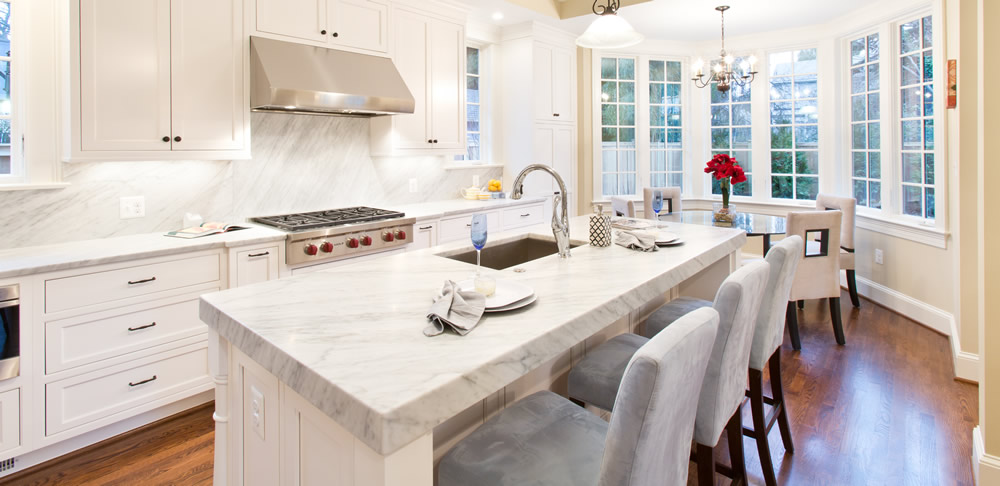The image portrays a bright, clean kitchen with a horizontally aligned rectangular frame. The kitchen cabinetry and ceiling are all white, contrasting with the darker brown wood tile flooring. Centered in the image is a marble-patterned rectangular island in shades of gray and white, featuring a sink with a visible tap, a wine glass with blue liquid, white ceramic plates, cloth napkins, and three cushioned gray chairs neatly pushed in.

To the left of the sink is a stainless steel gas stove with distinctive red knobs, flanked by three drawers with metal horizontal handles and upper cabinets with small circular knobs. On the far left of the image, there is a barely visible window, and another window is situated on the right side of the stove, which is complemented by a vent fan above.

In the background, a matching granite countertop runs behind the island, with additional cabinetry and a cooker. Beside the cooker lies a book, and above is an efficient vent system.

On the right side of the kitchen, a cozy breakfast nook is visible, featuring a round glass-top table surrounded by four white cushioned chairs with square cutouts in their backs and a flower vase in the center. This area is illuminated by natural light streaming through a series of six vertical rectangular windows, enhancing the airy and welcoming atmosphere of this well-organized, people-free kitchen.